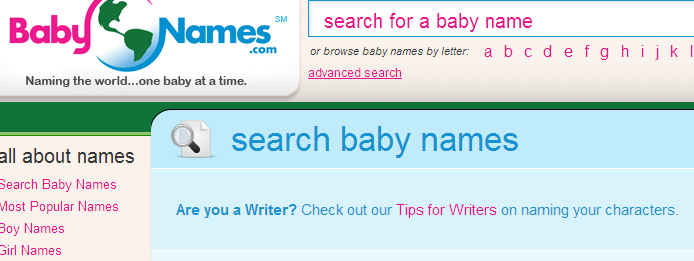This is a cropped screenshot of the BabyNames.com desktop website. In the top left corner is the Baby Names logo, featuring the word "Baby" in pink and "Names" in blue. Between these words is an image of a globe, displaying North and South America in green. The site’s tagline, "Naming the World One Baby at a Time," is prominently displayed beneath the logo. 

To the right of the logo sits a search bar with the prompt "Search for a Baby Name" in pink text. Directly underneath, there are options to search baby names alphabetically from A to L. Beside these options, there's a pink "Advanced Search" button.

A blue rounded-corner division below this contains the header "Search Baby Names" and invites users with the question, "Are you a writer?" followed by a clickable link in pink, "Check out our tips for writers on naming your characters."

On the left-side navigation pane, several website sections are listed, including "Search Baby Names," "Most Popular Names," "Boy Names," and "Girl Names." The background color for this navigation area is pink, matching the background of the alphabetical search section.